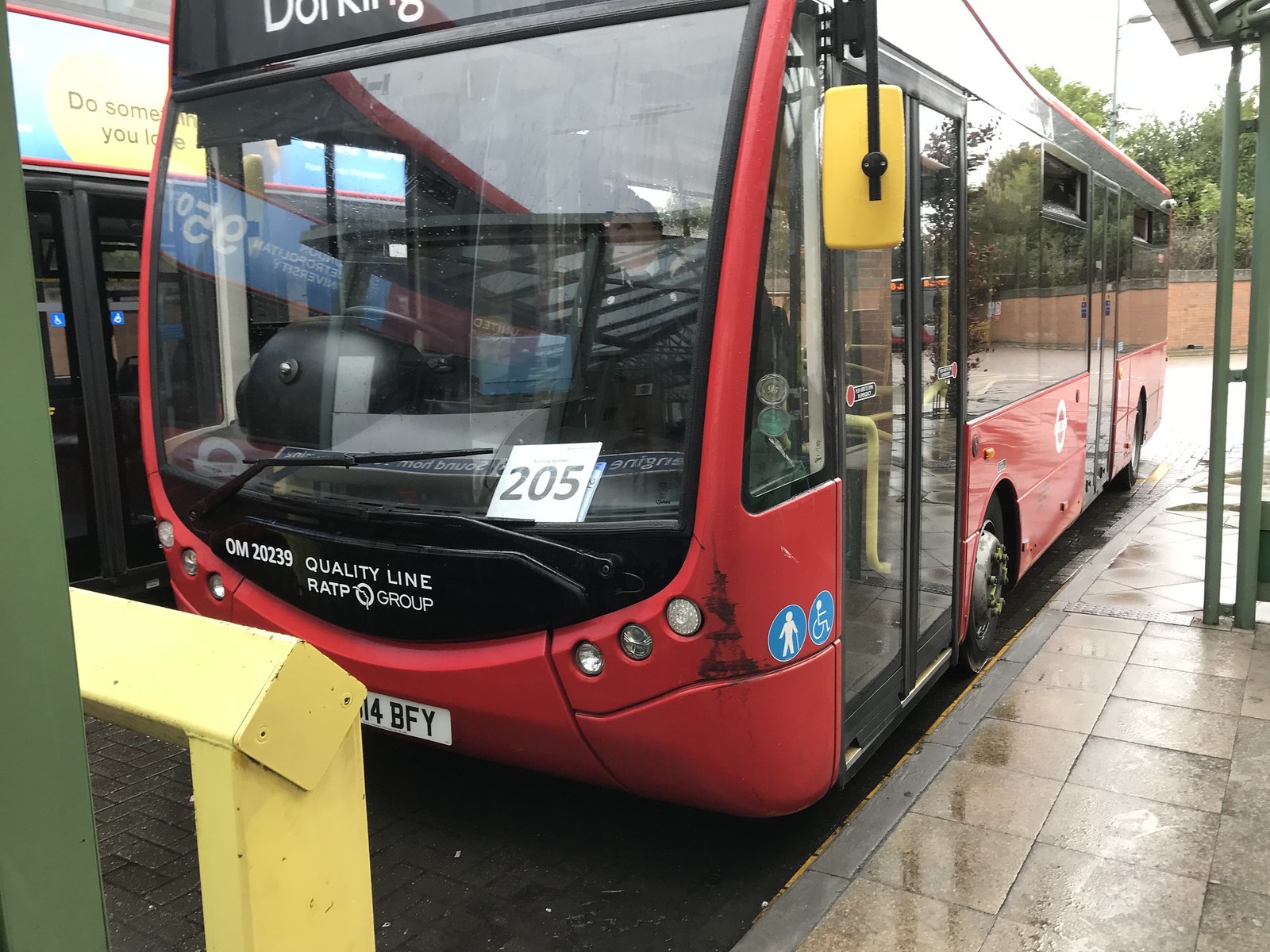The photograph depicts a red city bus, numbered 205, parked in a designated bus parking spot or possibly a bus station. At the front of the bus, a white sign with black letters indicates its number "205" and reads "Quality Line RATP Group." The bus sports a large windshield, and a visible window row along the side, with the top windows slightly open, possibly for ventilation. Though the windows are tinted, a driver might be faintly discernible inside. A yellow metal barricade in front of the bus suggests it can only reverse to exit. To the right of the bus, there's a bus stop or seating area, and nearby doors likely lead to a transit station. The ground appears wet, hinting at recent rain. The destination displayed on the bus starts with the letters "D-O-R-K".